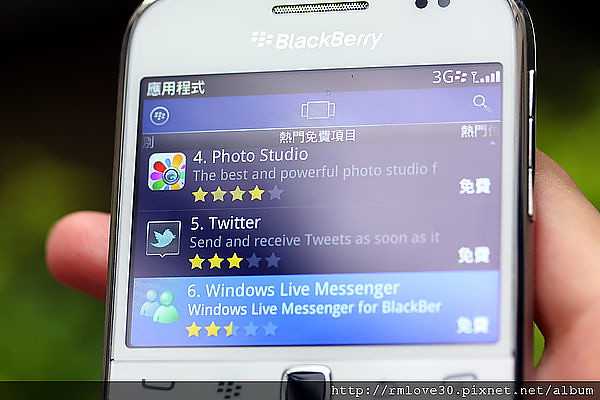The image is a close-up of a person's hand holding a white BlackBerry phone, with a partial view of the phone in the frame. The BlackBerry logo is prominently displayed at the top of the phone's screen, which is showing the app store. The apps listed include:

- Photo Studio, described as "the best and most powerful for all studio," rated four stars.
- Twitter, with the description partially visible as "send and receive tweets as soon as it," rated three stars.
- Windows Live Messenger, both the app and its rating of two and a half stars are visibly highlighted.

The BlackBerry phone indicates a 3G network connection with full signal bars in the top right corner. The background of the image is green and blurred, suggesting the photo was taken outdoors, possibly in a grassy area. Additionally, the bottom of the screen bears a URL: http://rmlove30.pixnet.net, which is partially visible. The overall scene evokes a nostalgic feel with the classic BlackBerry device being showcased in a relaxed, natural setting.